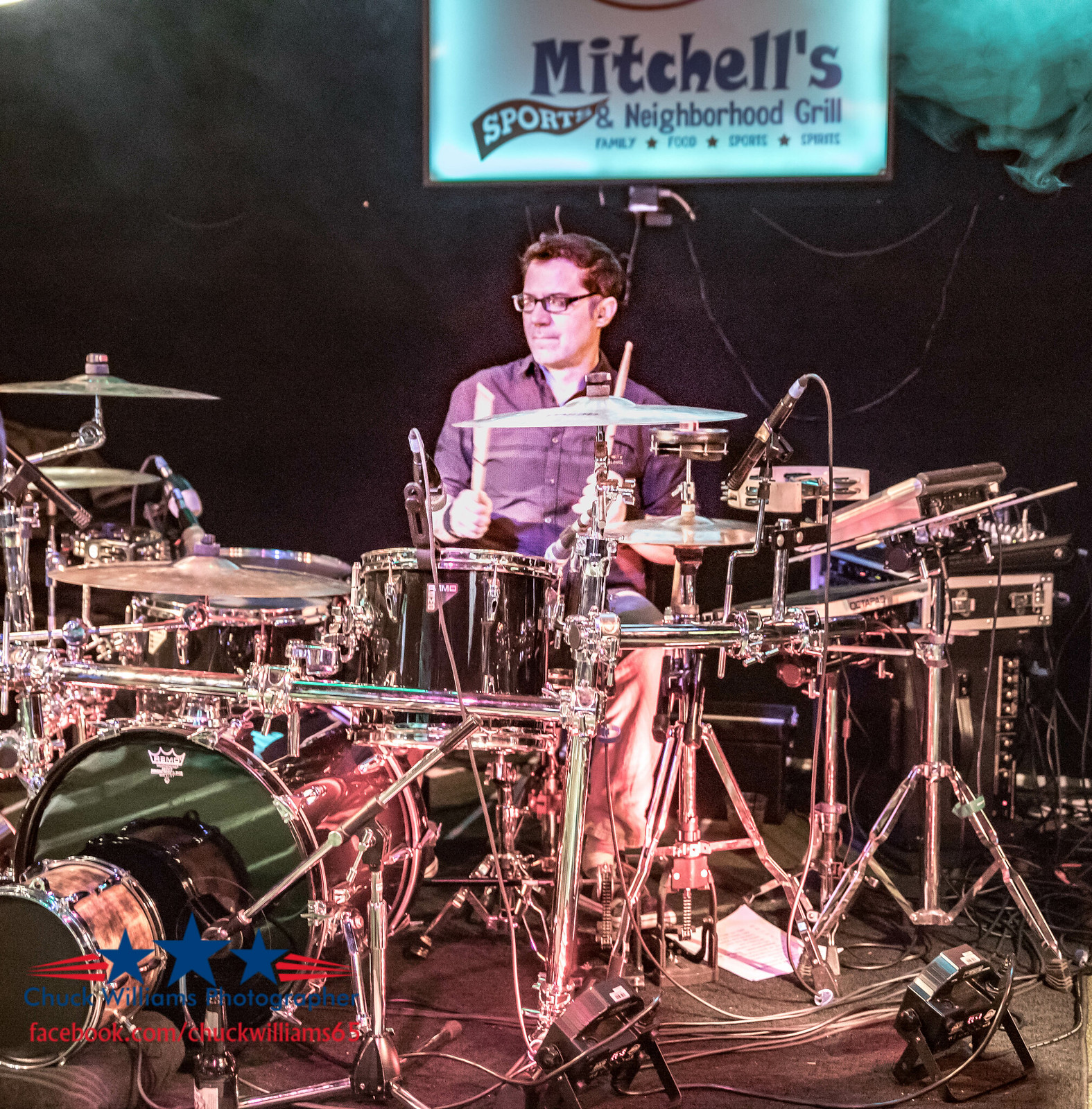The photograph shows a white male drummer with short, slightly wavy brown hair and black-framed glasses. He is captured mid-performance, seated behind an impressive and extensive drum set that envelops him. The drum set features glossy black drum heads and numerous components connected by super shiny chrome stands and bars, including holders for electronic equipment. The drummer is dressed in a purple buttoned-up collared shirt and khaki pants. The background is a solid black, contrasting sharply with a green smoky effect near the top of the image, possibly from a fog machine. A partially visible sign hanging from the ceiling behind him reads "Mitchell's Sports and Neighborhood Grill" on the bottom half, which also includes a red sports flag around the word "sports." The bottom left-hand corner of the image is marked with the photographer's credit in blue font, "Chuck Williams Photographer," followed by "facebook.com/ChuckWilliams65" in red font beneath it.